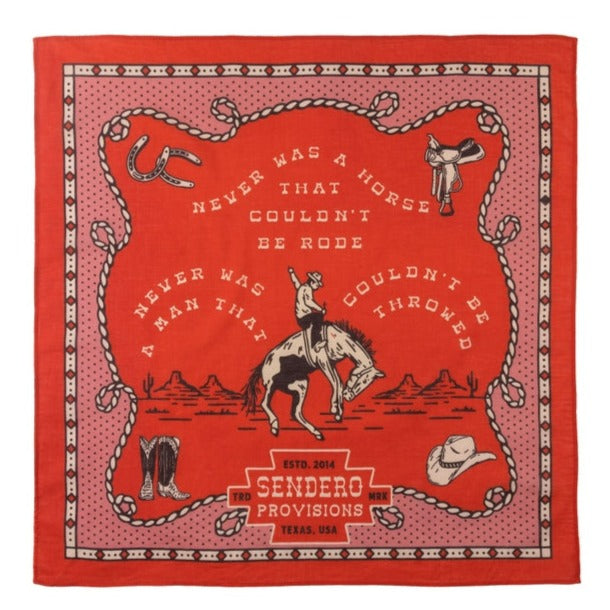This detailed caption combines the two descriptions into a coherent and comprehensive narrative:

"This is an image of a square-shaped poster with a vibrant red background. Right in the middle, there's a detailed black-and-white drawing of a horse in mid-buck, its head and back end pointing downwards, and a prominent hump in the center. A cowboy is depicted on top of the hump, attempting to ride the wild horse with one hand raised high in the air. Surrounding the central image is a motivational phrase written in white: 'Never was a horse that couldn't be rode. Never was a man that couldn't be throwed.' 

In all four corners of the poster, there are distinct thematic decals: two horseshoes in the upper left, a saddle in the upper right, a pair of boots in the bottom left, and a cowboy hat in the bottom right. A swirling rope artistically frames the central image and text, adding to the Western motif. 

Below the main composition, a banner reads 'Established 2014. Sendero Provisions, Texas, USA.' The background behind the rope is purple adorned with brown-colored dots. Enclosing this background is a white border decorated with orange stars, each punctuated by black dots, and the entire piece is further enclosed by a solid red border, completing the robust and lively design."